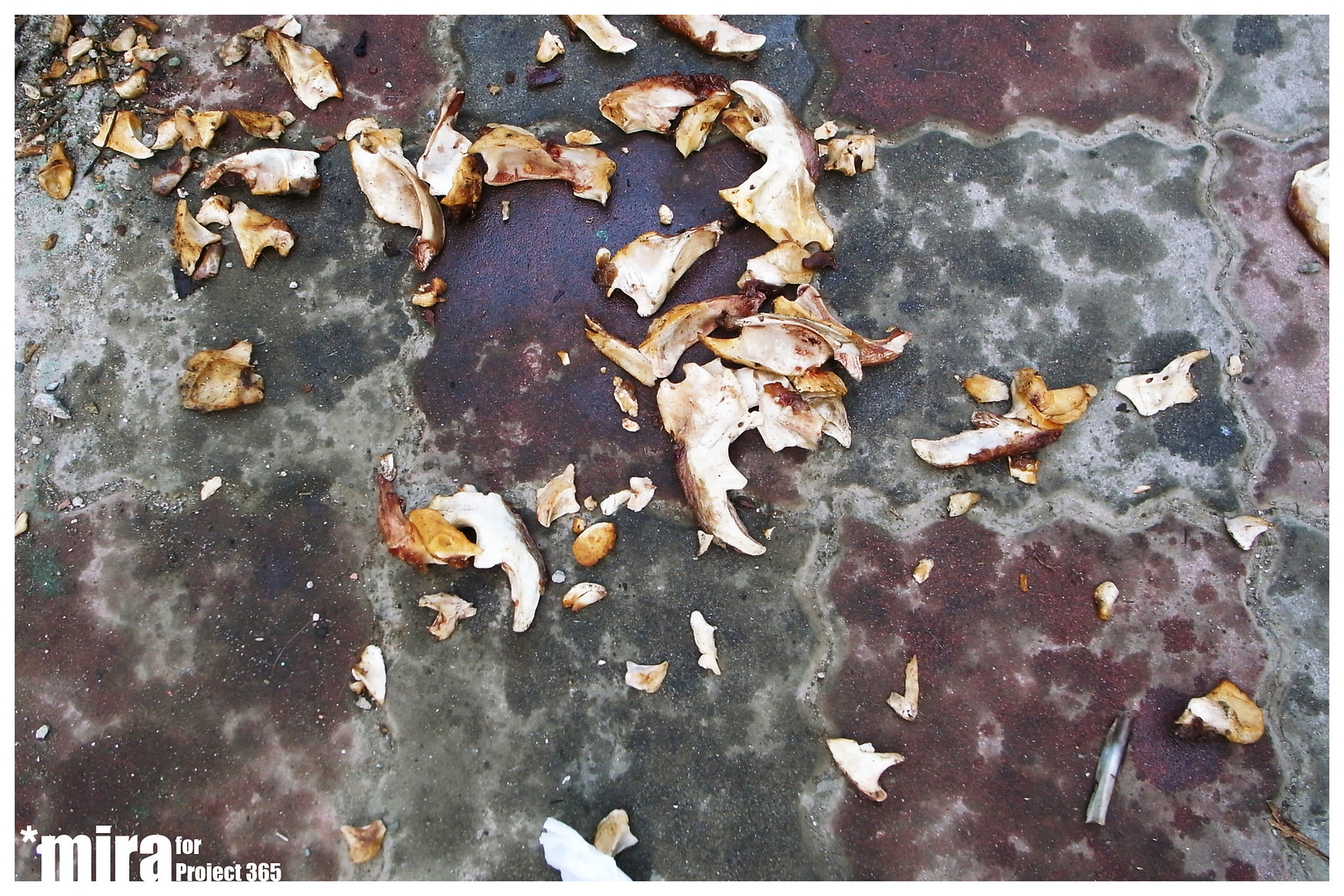The image depicts a tiled surface, possibly consisting of wet concrete, laid out in a checkerboard pattern with alternating colors of red, white, brown, yellow, and a few other hues such as an off-green, rust, and a touch of blue. The tiles have wavy, wiggly edges. Scattered all over the surface are broken pieces that resemble seashells or food peels, contributing to an overall chaotic and unclean appearance. The general scene looks like it may be related to some sort of environmental cleanup project, as suggested by the text in the bottom left corner, "M-I-R-A" along with a star symbol, indicating "MIRA for Project 365." The absence of people emphasizes the focus on the litter or debris, highlighting an urgent need for attention to the environment.